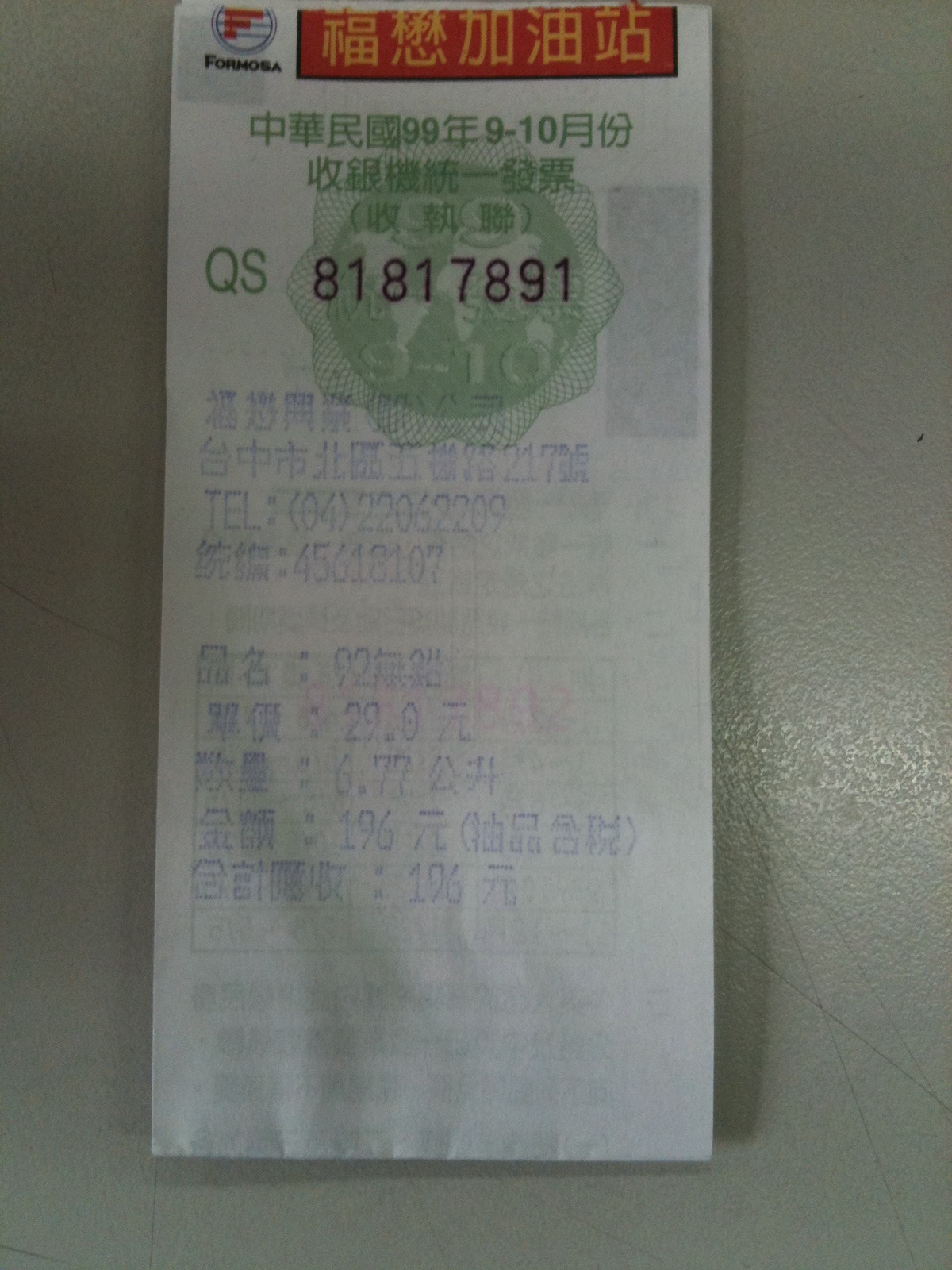The image showcases a receipt written in Taiwanese, featuring prominent Asian characters. At the very top, there is a striking red bar adorned with gold-colored characters. Centered below the bar is a circular emblem containing the word "Formosa" beneath a red letter "F." Positioned just below this emblem, there is a green stamp with Asian characters, followed by the letters "QS" in green, and next to it, the number "81817891" in black text. The receipt itself is white and exhibits faint blue ink printouts that presumably denote various monetary values. Additionally, a telephone number is visible at the top alongside numerous Asian characters scattered throughout. The receipt is placed on a white, textured surface that displays noticeable scratches.